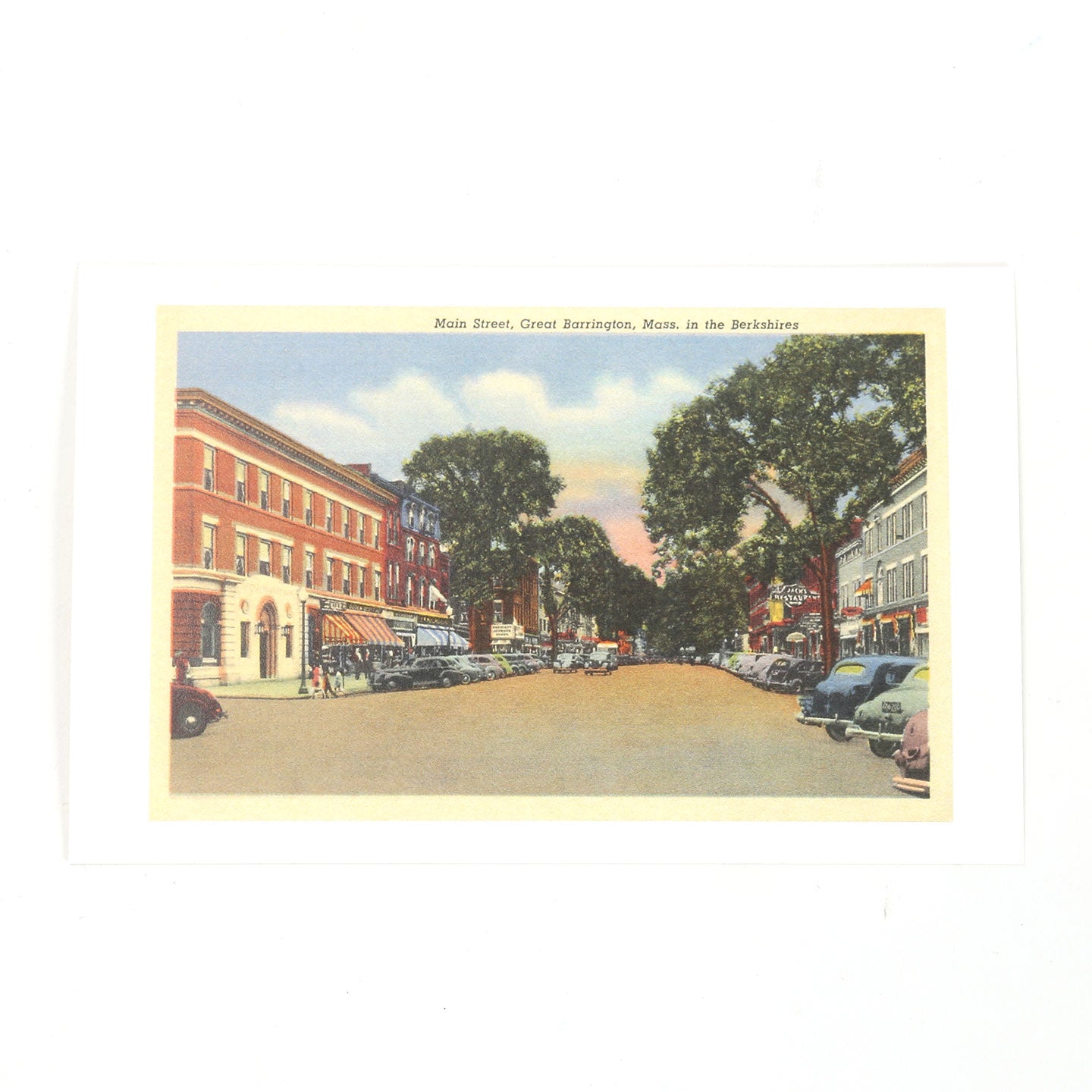This image appears to be a vintage postcard captioned "Main Street, Great Barrington, Massachusetts, in the Berkshires." The small, rectangular illustration or drawing, framed by a beige border, depicts a wide main street lined with cars from the 1940s or 1950s that are parked diagonally. On the left side of the street, there is a prominent red brick building with awnings, potentially a hotel and possibly a restaurant beneath the red awning. Adjacent to it, various storefronts continue down the street but are not fully visible. The right side features more buildings, including a notable two-story structure with a brick base and either gray or silver upper level. Tall trees line the street, adding a touch of nature to the urban scene, and a clear blue sky with fluffy clouds stretches overhead. Notably, the image shows no people, enhancing its nostalgic and tranquil atmosphere.